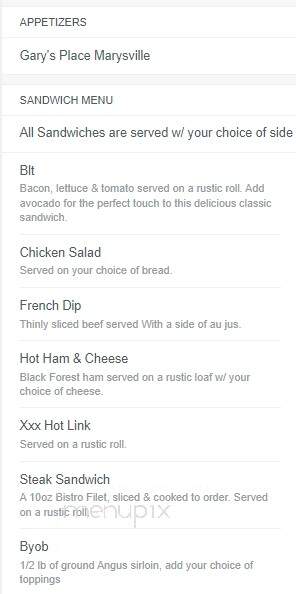This image is a screenshot in portrait mode, featuring a single long column against an off-white background. At the top, there is a light gray strip, followed by a section divided into two rows. The first row, on the left, has the word "APPETIZERS" in capital letters. Below this, the second row reads "Gary's Place Marysville."

Continuing down the column, there's another strip in a slightly off-white shade, after which the section titled "SANDWICH MENU" appears in all capital letters. Below this, another row informs that "All sandwiches are served with your choice of side."

The subsequent rows outline the sandwich offerings:

1. "BLT" - Bacon, lettuce, and tomatoes served on a rustic roll. An option to add avocado is available for enhancing this classic sandwich.
2. "Chicken Salad" - Served on your choice of bread.
3. "French Dip" - Thinly sliced beef served with a side of au jus.
4. "Hot Ham and Cheese" - Black Forest ham served on a rustic loaf with your choice of cheese.
5. "XXX Hot Link" - This item is somewhat ambiguous, labeled as "triple X hot link," and is served on a rustic roll.
6. "Steak Sandwich" - A 10-ounce bistro filet, sliced and cooked to order, served on a rustic roll.

Interestingly, there's a watermark reading "M-U-N-U-P-I-X" behind this section. The final row on the menu describes the "BYOB" (Build Your Own Burger) option, which includes a half-pound of ground Angus sirloin to which you can add your choice of toppings.